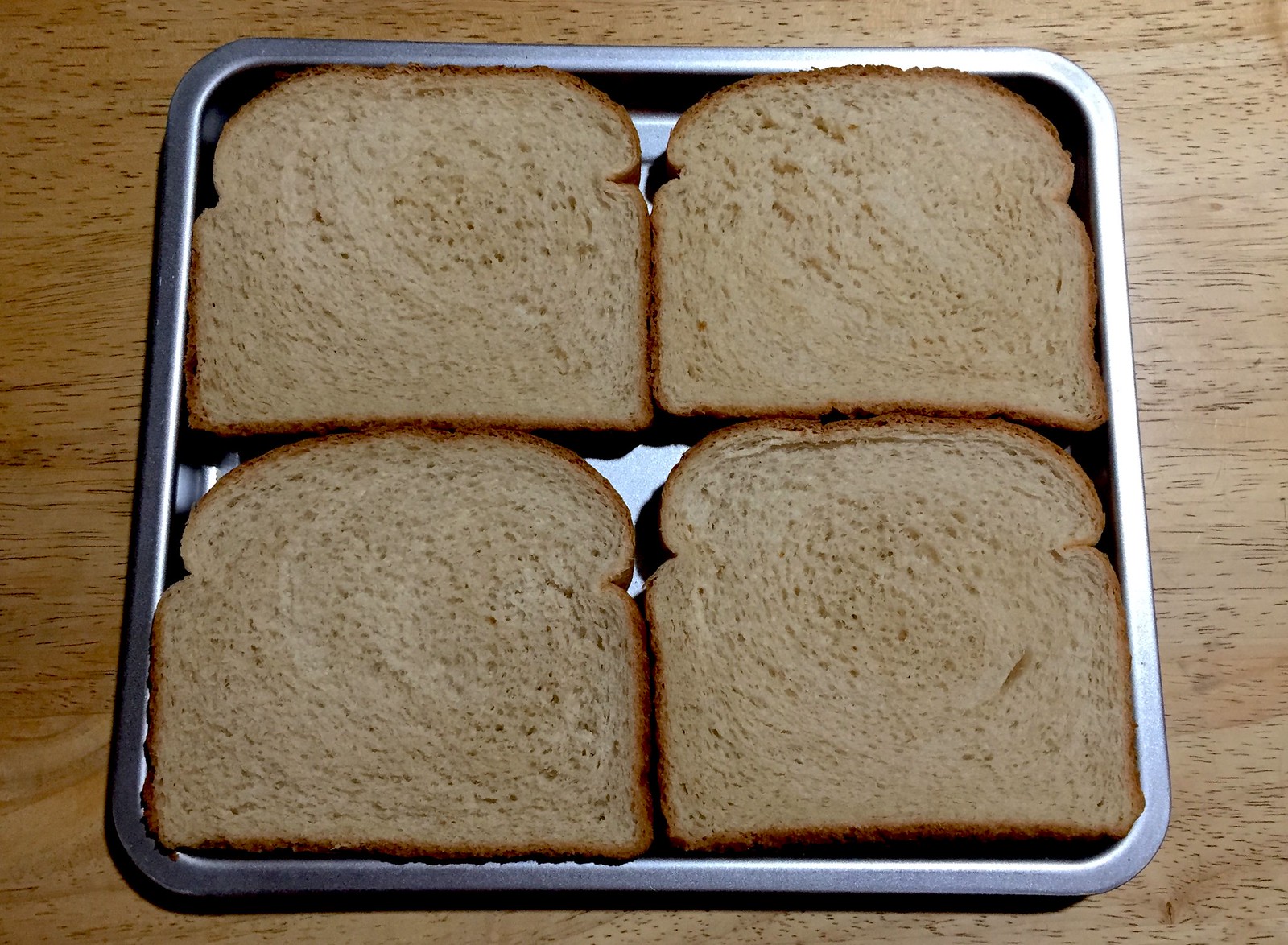This photograph captures a square, silver metallic baking tray placed on a light to medium brown wooden countertop or table. The tray contains exactly four slices of whole wheat bread, which neatly touch each other to form a tight square. The bread, characterized by its darker brown crusts and lighter brown interiors, blends almost seamlessly with the wooden surface in terms of color. Each slice is distinct in texture, but it's evident they all come from the same loaf. There's a tiny shadow on the left-hand side, hinting at an interior light source, but no noticeable text or details that distract from the simplicity of this domestic scene. The subtle gaps where the crusts’ rounded edges meet create a faint V shape, adding a touch of detail to the arrangement.